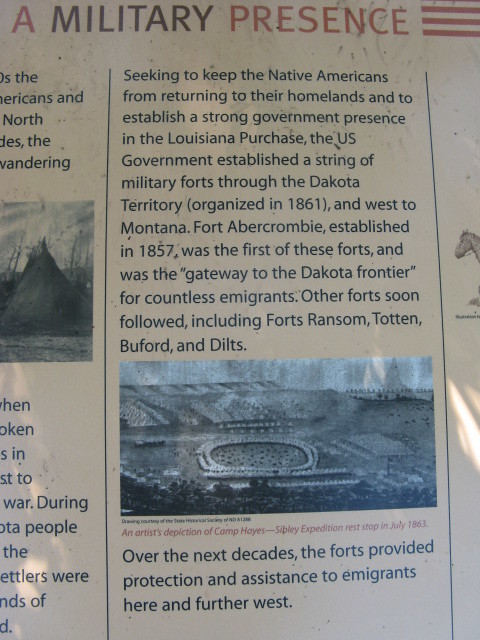This is a clipping, possibly from a newspaper or magazine, that details historical military efforts to establish a strong government presence in the Louisiana Purchase and deter Native Americans from returning to their homelands. It features a headline in both black and red text that reads, "A Military Presence." A passage on the left side explains that to accomplish these goals, the U.S. government established a series of military forts throughout the Dakota Territory, west to Montana, starting with Fort Abercrombie in 1857. This fort served as the gateway to the Dakota frontier for countless emigrants. Other forts quickly followed, including Forts Ransom, Totten, Buford, and Diltz. Over the next decades, these forts provided crucial protection and assistance to emigrants traveling both here and further west.

The image shows an artist's depiction of Camp Hayes, a rest stop for the Sully Expedition in July 1863. This illustration, inaccurately assumed to be a photograph at first, captures the historic essence of the site. Additionally, a partial image of what appears to be a horse is visible on the right side, further enriching the historical context. The clear black-and-white background of the text makes the historical narrative stand out vividly.